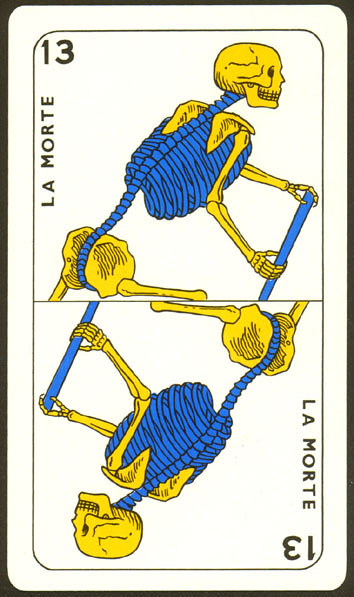This image features a card with a striking visual design. The card itself is framed by a black outer border, which contrasts sharply with the predominantly white interior. The central focus of the card includes artistic illustrations divided into two mirrored halves—one upright and the other inverted.

On the top half of the card, the word "La Monte" is inscribed on the left side, accompanied by the number "13" prominently displayed in bold at the top. The central figure within this section is a human skeleton depicted with a unique color scheme: a blue spine and ribs, yellow shoulders, arms, hips, thigh bones, and skull. The skeleton is holding a blue staff-like object in its hand.

The bottom half of the card mirrors the top half but in an inverted orientation. This reflection shows the same skeleton with yellow thigh bones, blue spine and ribs, yellow shoulders, hands, and skull. The inverted skeleton faces left, with its back on the right side, holding the blue staff on the right. The detailed and vibrant illustration provides a visually engaging and symbolic depiction, making this card particularly intriguing.